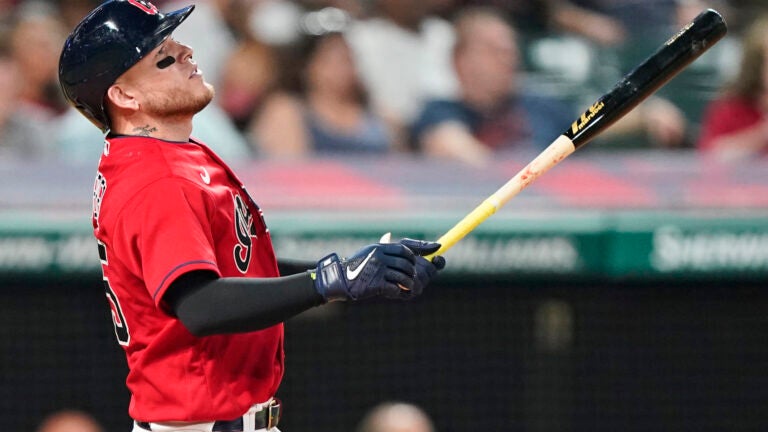In this highly detailed, photographic-style image set outdoors in a ballpark, a baseball player—a white or Hispanic male—is captured in a dynamic profile shot as he prepares to bat. His focused gaze is directed upward, possibly tracking the ball he has just hit or is about to hit. He dons a black Cleveland Indians helmet adorned with a red "C" logo, complemented by a red jersey showcasing part of his number on the back, notably the number 5. Underneath his jersey, he wears a long black-sleeved shirt. 

The player grips a Marucci baseball bat, its design featuring a blend of light wood and black, with the handle distinctly marked in white. His hands are protected by black Nike batting gloves, and he's dressed in white baseball pants cinched with a black belt. 

In the blurred background, the top of a green dugout is visible, along with indistinct spectators populating the stands. Among the out-of-focus crowd, a man and a woman, both appearing to be white, can be partially discerned, with the woman having black hair. The scene captures a moment steeped in the anticipation and energy of the game.